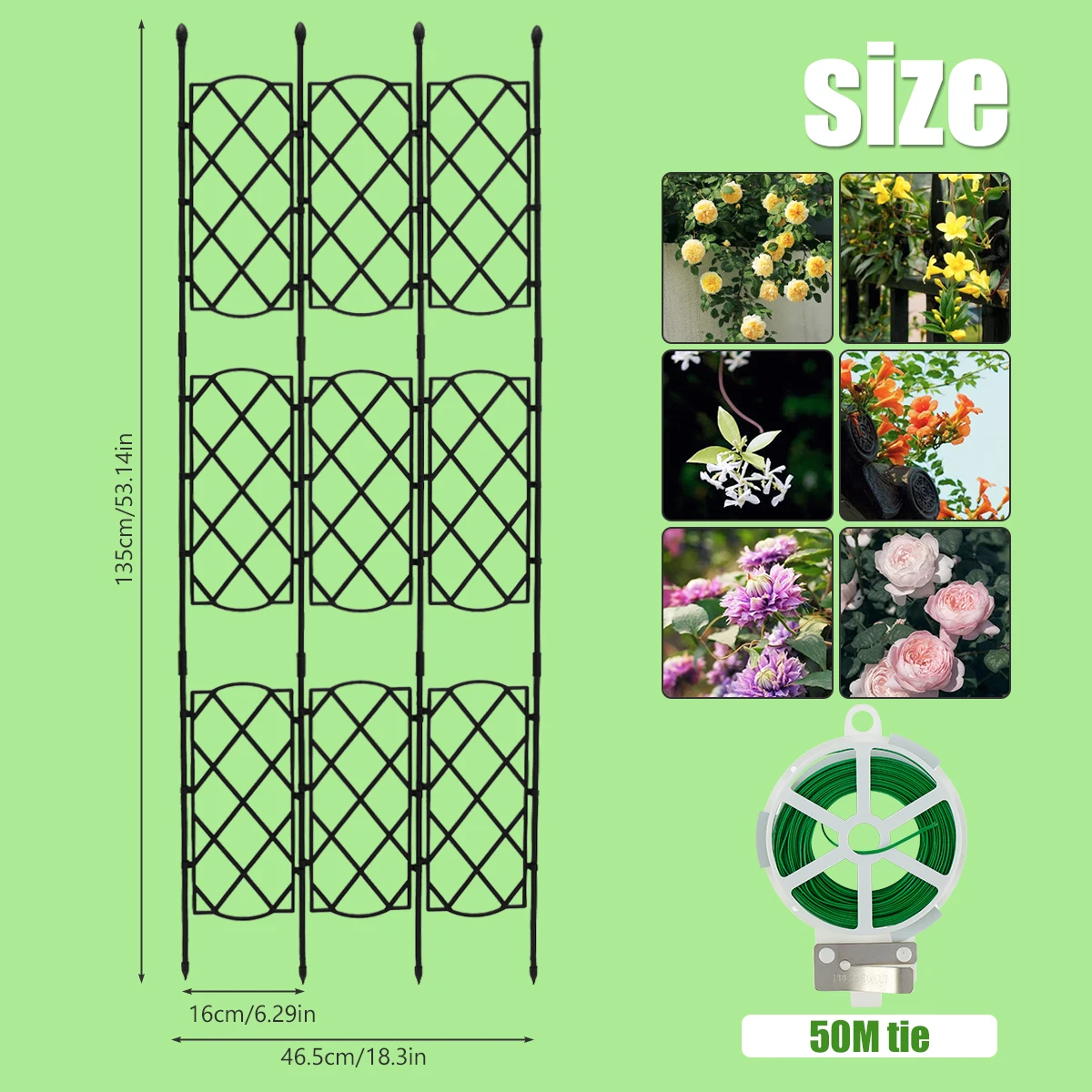This image is an advertisement for a garden trellis, set against a light green background. The ad features a schematic on the left side illustrating the trellis structure with detailed dimensions: it stands 135 centimeters (53.4 inches) tall and 46.5 centimeters (18.3 inches) wide, with each section between the poles measuring 16 centimeters (6.29 inches). The trellis comprises four black poles connected by diagonal crisscross panels arranged in three levels.

On the right side of the ad, there are several small photographs showcasing different types of flowers that can be grown on the trellis. These examples include two varieties of climbing roses (one yellow and one pink), tall lavender bee balm flowers, climbing jasmine, trumpet flowers, and another yellow climbing vine.

Prominently displayed at the bottom right of the ad is an image of the product—a green spool of wire tie, labeled "50m tie." The word "size" is written clearly in large white letters across the image, emphasizing the dimensions and the utility of the trellis for gardening.